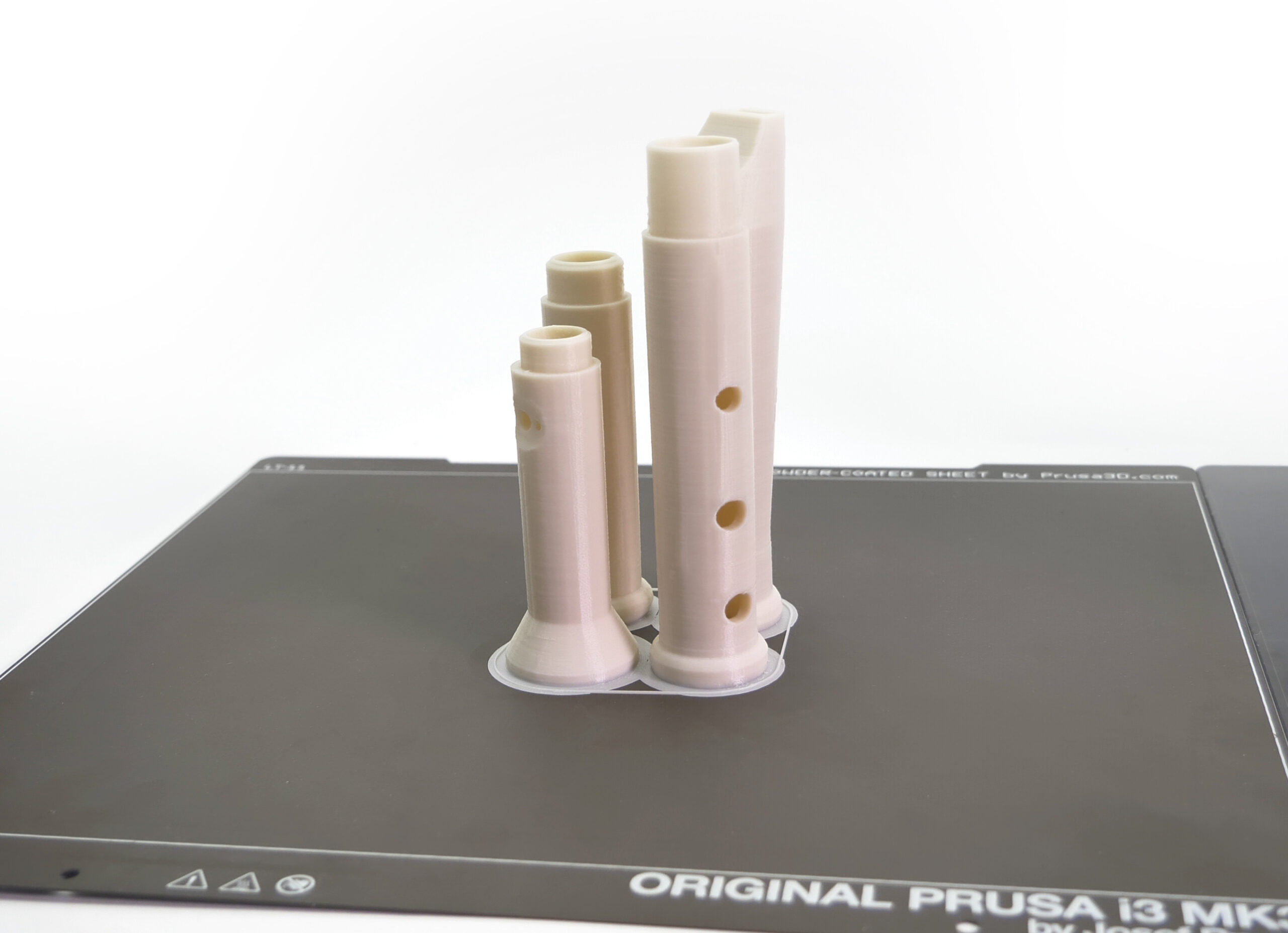The photograph features a detailed composition of four cylindrical components displayed on a dark gray mat labeled "Original Prusa i3 MK3" in white text. These objects, primarily light pink in color, bear a resemblance to hair curling hot rollers but with an added touch of beige, evoking the appearance of flute segments. Each cylinder varies subtly, with one featuring visible holes, akin to finger holes on a flute, while the others seem designed to interconnect without such perforations. The meticulously arranged items are showcased on the mat, enhancing their prominence against the clean, white background. The image's compelling contrast and focus on the delicate pink hues against the dark gray surface beautifully highlight the unknown purpose of these intriguing components.